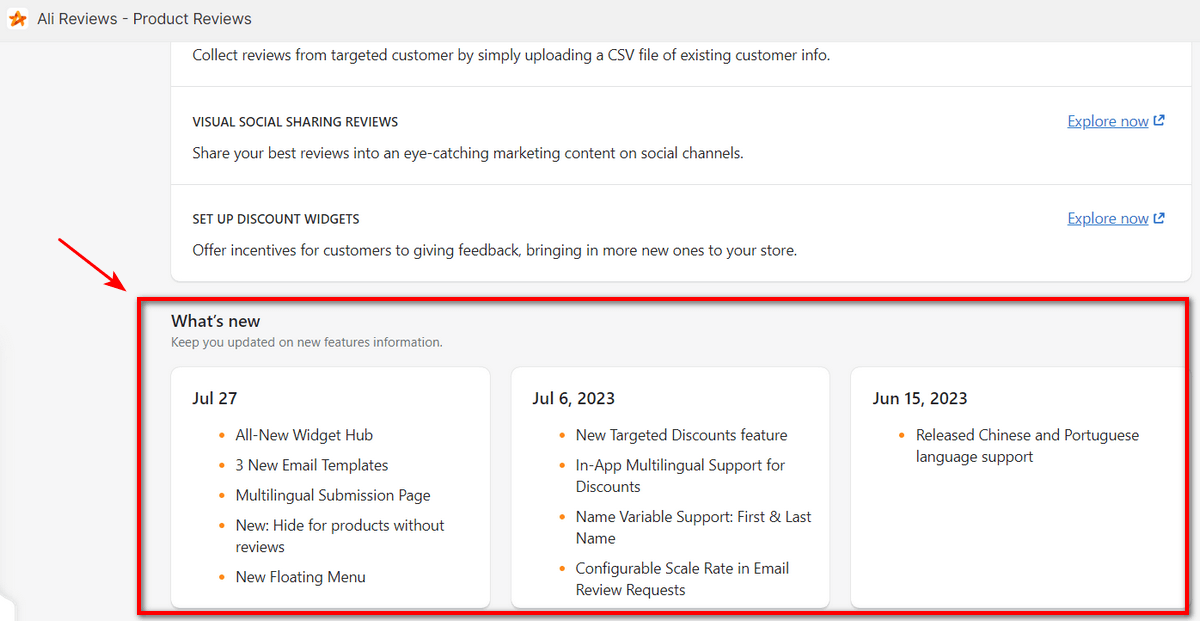This is a rectangular screenshot of a review website titled "Alley Reviews - Product Reviews," displayed in black text. On the far left of the image, there is a star-shaped icon filled with yellow, orange, and red hues against a white background. The main portion of the screenshot features a light gray background with several squares of information, each set against a white background. 

The text within these squares is predominantly black. Various categories are listed throughout the image. A notable feature is a red arrow pointing towards the lower section, which is outlined by a red border. This section is labeled "What's New" in black text, followed by a gray subtitle that reads, "Keep You Updated on New Features and Information." 

Within this highlighted section, there are three square-shaped areas with white backgrounds, each containing black text and dated entries: July 27th, July 6th, 2023, and June 15th, 2023. Additionally, there are circular orange bullet points marking different topics.